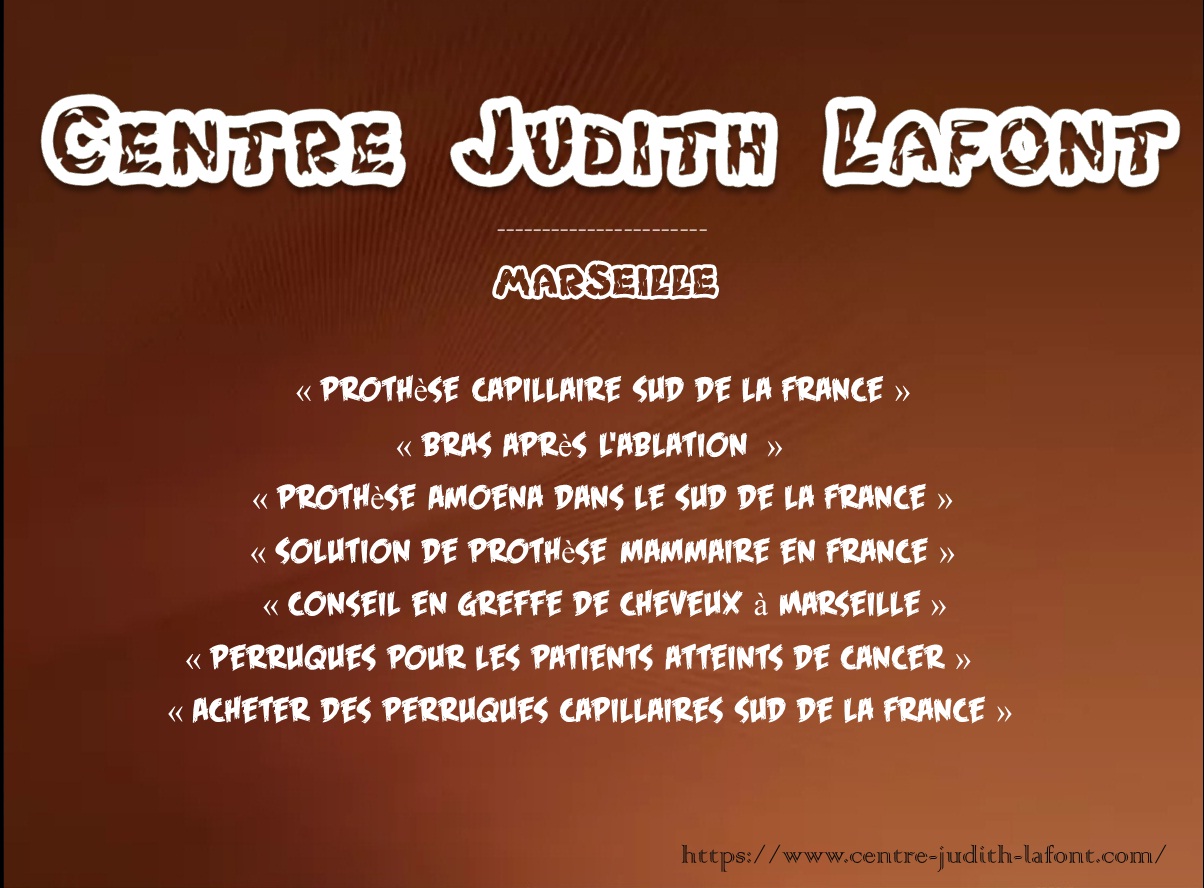The image appears to be an advertisement with a brown gradient background that transitions from a dark brown on the upper left to a lighter brown on the bottom right. At the top, in large white font, it reads "Centre Judith LaFont", with "Centre" spelled in the British English style. Under this, there is a dotted and dashed line followed by the word "Marseille". The text is centrally aligned and spans the middle of the image. The image contains seven French sentences beneath the main title. Additional details include various arrows, likely associated with each sentence. In the bottom right corner, there is a website URL in smaller black text: https://www.centre-judith-lafont.com. The overall aesthetic features a pleasant font and evenly distributed text, all within the cohesive colour scheme.